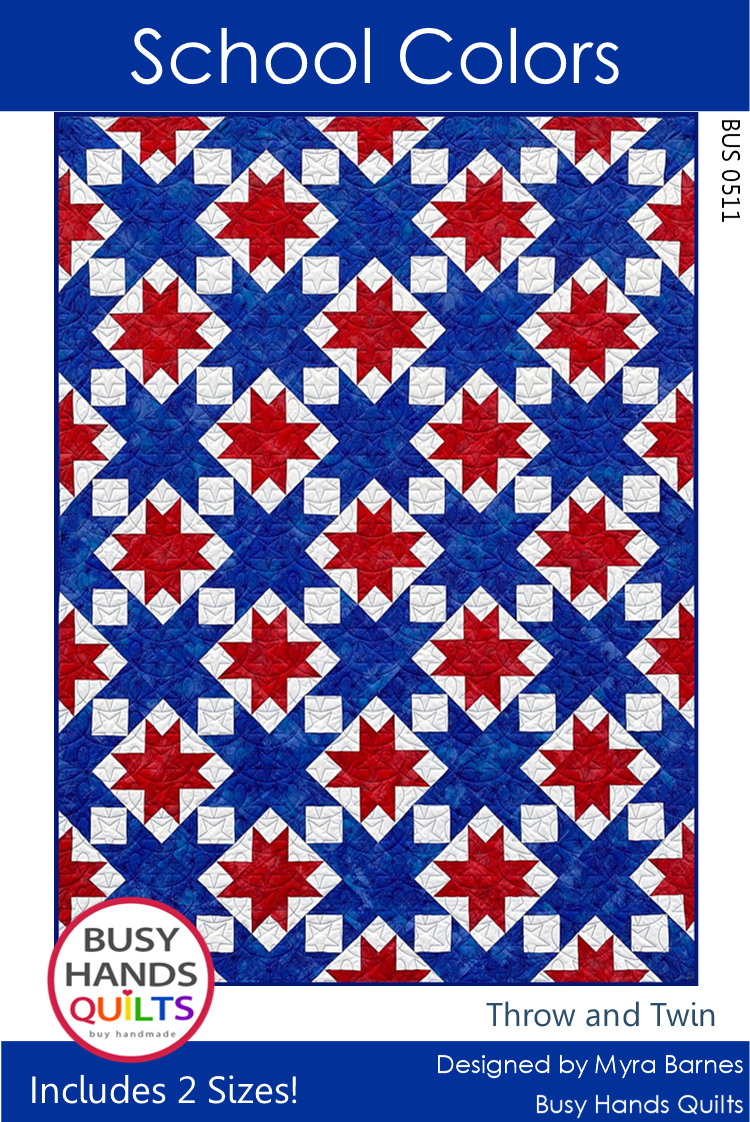The image titled "School Colors" prominently features a blue background with a flag-like pattern. At the top, a horizontal blue rectangle contains the title. The central part of the image displays a blue vertical rectangle adorned with neat diagonal lines of white diamonds and squares. Each white diamond contains a red cross with its tips truncated, creating a distinctive design. The red crosses resemble a maple leaf or double-cross star pattern. In the lower left corner, a red circle bears the inscription "Busy Hands Quilts by Handmade." Adjacent text in blue and white reads "includes two sizes!" along with "throw and twin designed by Myra Barnes, Busy Hands Quilts." An additional vertical inscription on the side reads “bus 0511.”